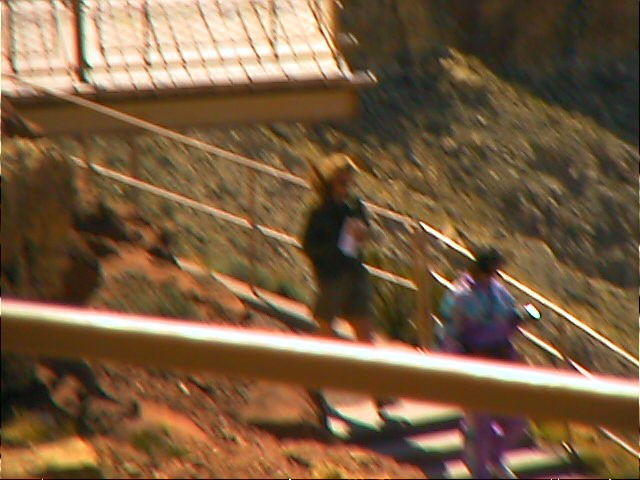This photograph, with its retro orange hues, features a blurry scene of two individuals descending a staircase. The image's prominent blur and nostalgic color palette evoke a vintage aesthetic. The staircase itself, adorned with a metal handrail, is mirrored by another metal rail crossing the lower third of the image, partially obscuring the individuals. This positioning suggests the photographer is likely capturing the scene from another set of stairs, possibly part of the same spiraling structure. In the background, to the right, a patch of grass is visible, while the center showcases a collection of orange-tinted rocks. Adding to the composition, a building with a metal roof appears in the top left corner, completing the intricate and layered perspective of the photograph.